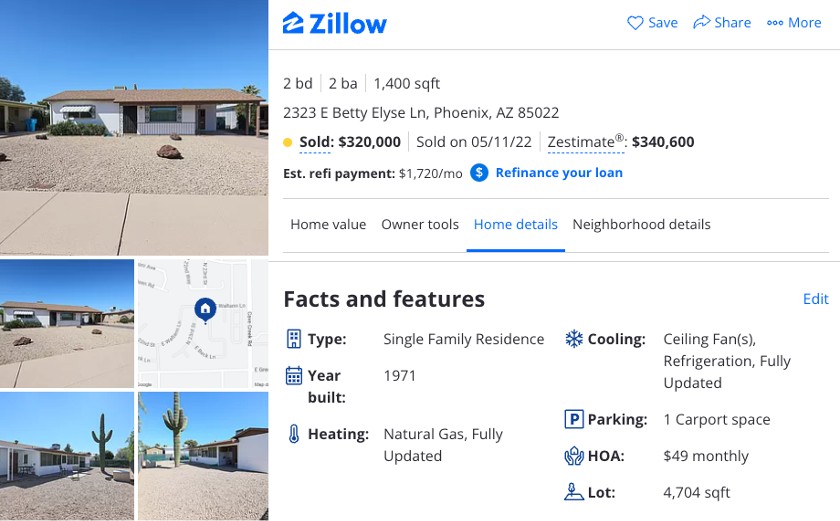**Detailed Description of Zillow Listing Screenshot**

This screenshot from Zillow presents a detailed overview of a single-story house that was recently listed. The primary image on the left showcases the front of the house, featuring a metal awning above the entrance and a carport. The front lawn is landscaped with gravel, punctuated with several red lava stones.

Below the main image are four additional photos. The upper left and two bottom images display various exterior views of the house, including two that capture the backyard area. Notably, the backyard is also covered in gravel and is dominated by a towering Saguaro cactus. The upper right image is a map showing the house's location.

At the top right of the screenshot, there are interactive options including "Save," "Share," and "More." Below these options, brief detail results for the house are provided: it is a two-bedroom, two-bathroom home with 1,400 square feet of living space. The house's address indicates it was sold for $320,000 on May 11, 2022. Zillow's estimate of its market value is between $346,000 and $340,600. Additionally, the estimated monthly refinancing payment for this house is $1,720.

The detailed section titled "Facts and Features" reveals the following:
- **Type:** Single-Family Residence
- **Year Built:** 1971
- **Heating:** Natural Gas
- **Cooling:** Fans and Refrigeration
- **Parking:** Carport with one spot
- **HOA Fee:** $49 per month
- **Lot Size:** 4,074 square feet

This detailed information provides a comprehensive view of the house's features and its financial details, allowing potential buyers to make an informed decision.